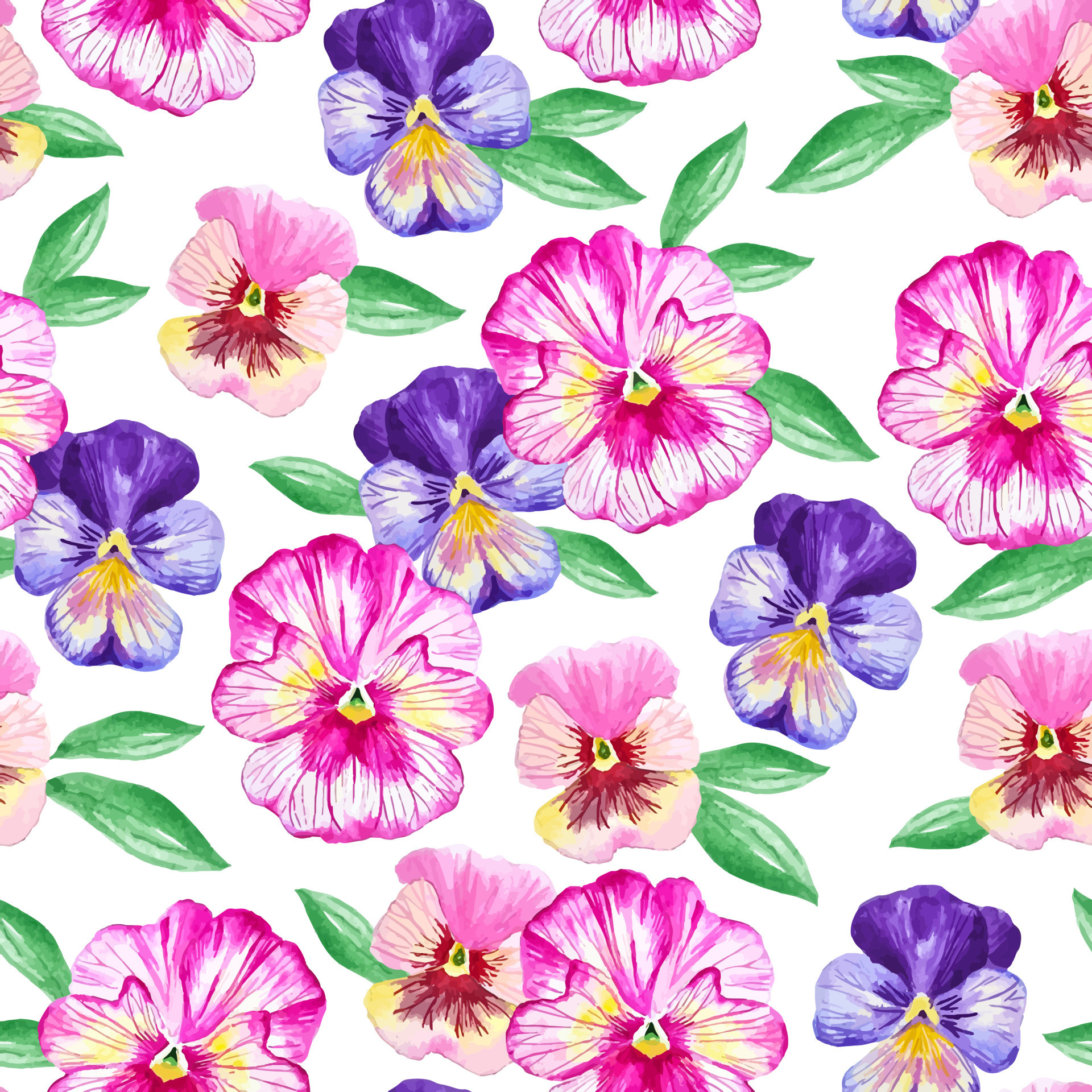The image is a meticulously detailed art print, designed with a careful blend of watercolor and digital techniques. Set against a crisp white background, various vibrant flowers including pinkish-white hibiscuses, deep purple and lavender African violets, and peach-colored flowers with red centers, are evenly scattered across. Among them, smaller white flowers provide delicate accents. Green leaves, varying in size, accompany the flowers, contributing to an overall symmetrical and balanced aesthetic. Some of the flowers, like the hibiscuses and African violets, feature splashes of yellow near their centers, adding a touch of brightness. The print's arrangement gives it a seamless, wallpaper-like quality, making it visually appealing and richly illustrative.